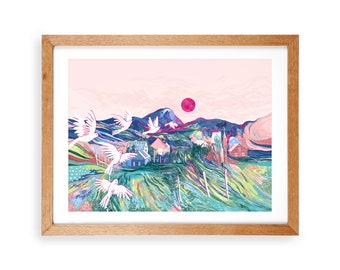The framed artwork in the image is a detailed landscape painting within a wooden rectangular frame. The frame itself is a light shade of brown with a white border just inside it, enhancing the focus on the painting. The painting primarily features a mountainous region depicted in dark indigo and blue hues, with white-tipped peaks suggesting the presence of snow. In the sky above the mountains, there is a magenta-colored sun, and the sky itself transitions through shades of red, peach, and light pink, creating a dramatic and serene backdrop. 

In the foreground, the landscape includes green and yellow grassy areas. Off to one side, there is a house nestled among some trees, their trunks distinctly rendered. Additionally, the painting is graced by six white birds, which appear to be flying in formation from the left side towards the middle of the painting, contributing to the dynamic composition of the piece.